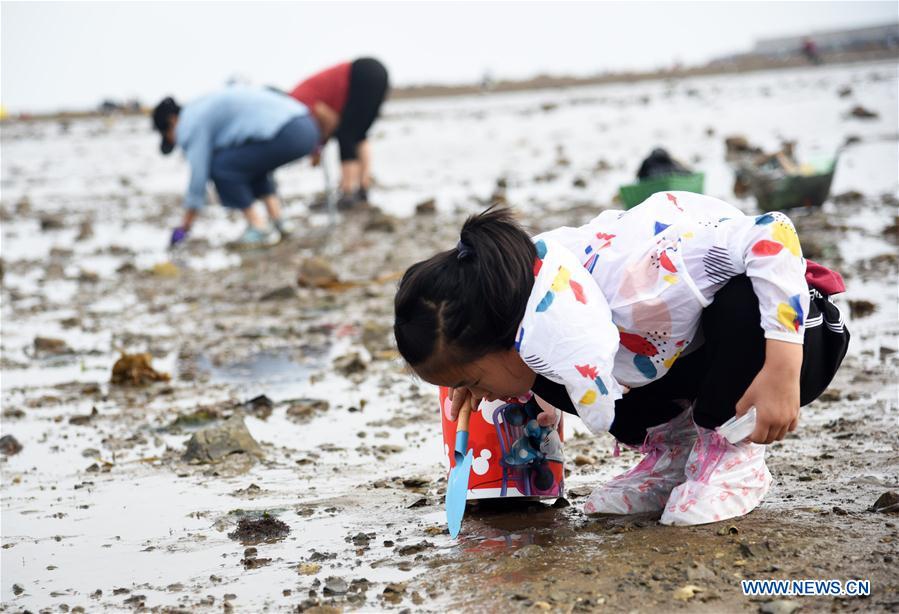This image captures a family of three engaging in beachcombing activities on a muddy, wet surface that appears to be a tidal flat. Central to the image is a young girl, positioned slightly to the right, intently digging into the sand with a blue hand shovel. She is dressed in a geometric-patterned white raincoat featuring blue, yellow, and red designs, paired with black pants and white-and-pink shoes. Her dark hair is tied back in a ponytail. Next to her is a red bucket adorned with Mickey Mouse logos, and she holds a small, clear plastic container in her other hand, possibly inspecting for small marine creatures.

In the background, slightly out of focus, are two adults, presumably her parents, also bending down and searching the sand. The father is noticeable in a light blue jacket and blue pants, while the mother wears a red T-shirt and black pants, both equipped with tennis shoes. Although the trio hasn't found anything yet, their engrossed activity suggests optimism in their search. Marking the image in the bottom right corner is a blue watermark reading "www.news.cn."